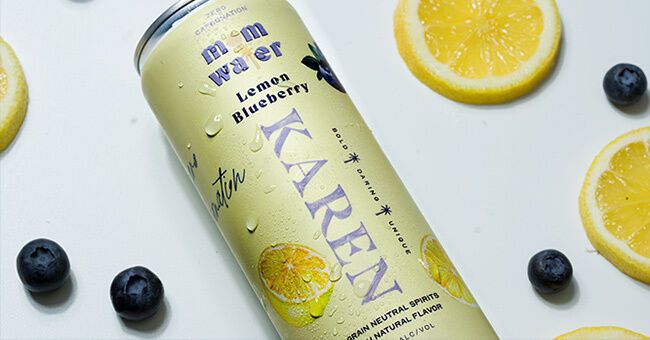This image depicts a close-up shot of a tall, slender can of a beverage titled "Mom Water." The can, set on a white surface and positioned horizontally in the middle of the image, features a light yellow background. At the top of the can, the words "Mom Water" are prominently displayed in blue text, with the 'O' and 'T' subtly highlighted in light yellow. Below that, "Lemon Blueberry" is written in black letters, referencing the flavor of the drink, which also contains "Grain Neutral Spirits All Natural Flavor," indicating it is an alcoholic beverage. Running vertically down the side of the can is the name "Karen" in light purple text. The chilled can, evidenced by visible water droplets, is surrounded by various fruit illustrations and real fruit pieces on the surface. These include heavily cut lemons and scattered blueberries: to the left and right of the vertical text "Karen" on the can, lemon slices and blueberries are positioned. Additionally, on the white surface, there are two more blueberries and a lemon slice visible near the top left, and another lemon wedge to the top right, with an additional blueberry nearby.